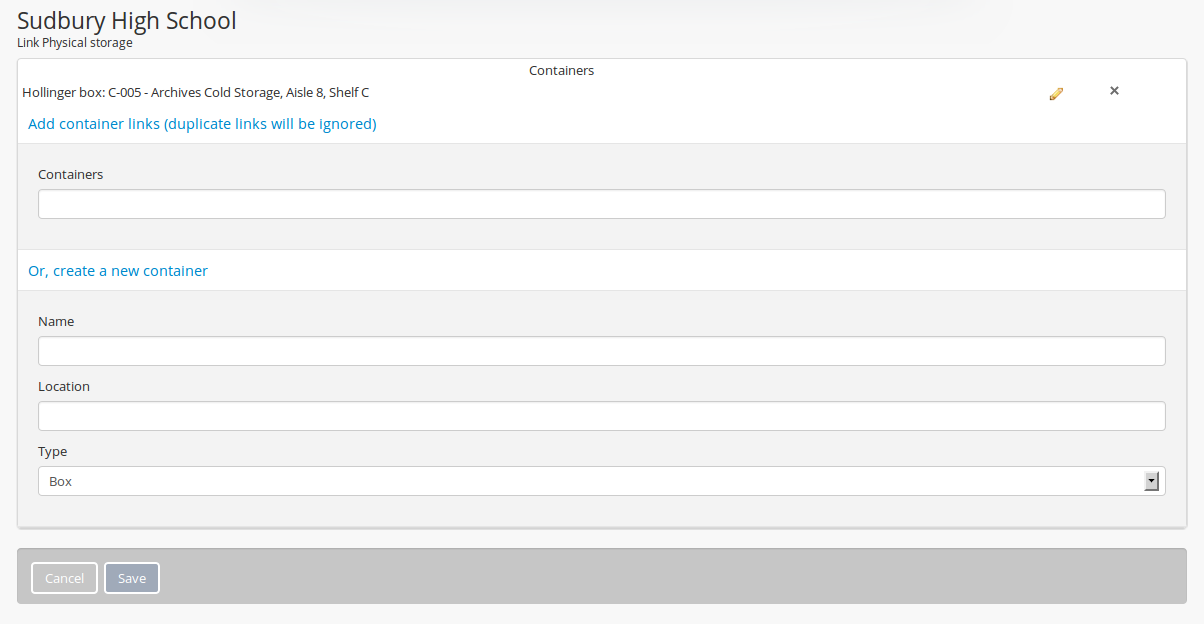The image displays a sophisticated application interface designed for linking physical storage locations to a specific school, identified as Sudbury High School, as mentioned in the top left corner. Below this, there is a heading labeled "Link Physical Storage". The application provides functionality to add container links using a pencil and tool icon. Users can specify existing containers or create new ones by inputting a name, location, and type for each container. There's a hyperlink indicating that duplicate container links will be ignored to prevent redundant entries.

The interface includes dropdown menus for selecting container types, although the specific options available in the dropdown are not visible in the image. In the bottom left of the screen, there are "Save" and "Cancel" buttons, allowing users to either save their entries or cancel the operation if they choose not to proceed. The overall purpose of the application is to create and manage storage locations efficiently, enabling users to keep accurate records of where various items are stored, which can be particularly useful for organizing resources within the school.